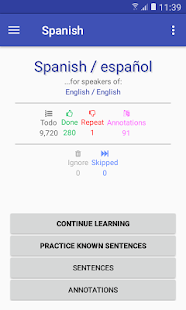The image depicts a screenshot from a mobile app, showcasing various interface elements. At the top of the screen, there is a purple-colored border. Within this border, on the top right side, there are icons indicating full Wi-Fi signal, cellular data with three or four bars, a full battery icon in white, and the time displayed as 11:39. Just below this border, in a slightly lighter purplish-blue color, is the word "Spanish" written in white text. To the left of this text are three vertical lines, and to the right are three vertical dots.

Beneath this section, within a white area, there is blue text that reads, "Spanish / Español for speakers of English / English." A gray line divides this part of the screen. Below the line, it indicates "Total 9720," accompanied by icons showing a thumbs-up with "Done 280," a thumbs-down with "Repeat 1," "Annotations 91," "Ignore 0," and "Skipped 0."

At the bottom of the screen, there are four gray blocks. The first block is labeled "Continue Learning," the second is "Practice Known Sentences," the third is "Sentences," and the fourth is "Annotations." The labels "Sentences" and "Annotations" are displayed in a slightly lighter and less bold font compared to "Continue Learning" and "Practice Known Sentences."